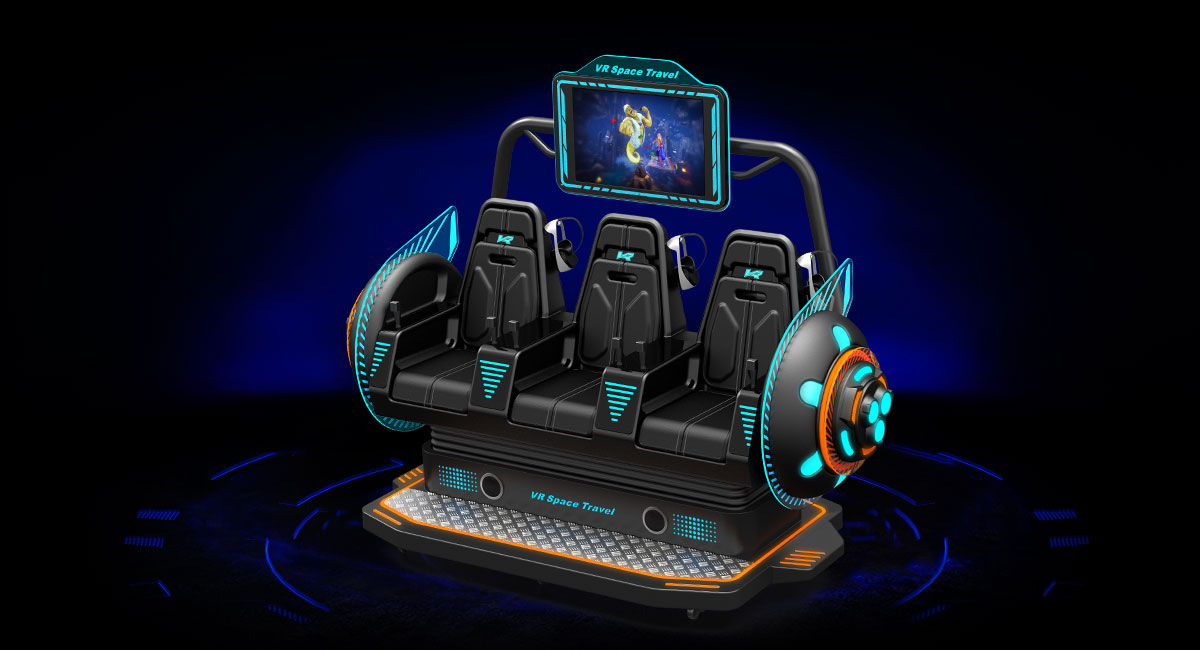The image depicts a detailed rendering of an amusement park ride designed to simulate a VR space travel experience. The setup features three black, high-backed chairs with firm foam cushions, arranged side-by-side and separated by solid armrests. The chairs are situated on a heavy steel base with a diamond-cut, non-slip metallic pattern for traction. Blue neon lights decorate the sides and arms of the chairs, extending down to the floor, while additional green trim with electric parts adds to the futuristic aesthetic.

Each seat has a circular dial on either side, suggesting potential swivel or rotation capability. Above the chairs, a bar supports an LCD screen that prominently displays the title "VR Space Travel" alongside an animated cartoon, seemingly of a genie emerging from a lamp. The floor features a bubbly, textured pattern illuminated in orange and red lights, with the text "VR Space Travel" lit up in blue at the base.

Beside each chair, there is a hook holding a VR headset, solidifying the ride's immersive purpose. The overall scene is set against a blue background, rendered with medium to low-grade CGI, incorporating a mix of bright blue and orange graphics for added visual appeal.